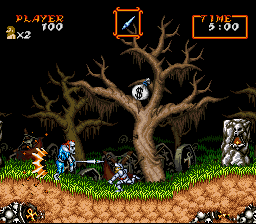This is a screenshot from an older or retro-styled point-and-click video game. The scene is set in a dark and eerie graveyard, characterized by a stark black background. Central to the image are two large, leafless trees, one with Spanish moss hanging from its crooked, pointy branches. In one of the trees, there's a conspicuous money bag.

The ground is a layered mix of green grass and earth with caverns visible beneath, filled with skulls and stones. Scattered throughout the scene are several gravestones, some with crosses.

Two characters are in mid-action, seemingly engaged in a fight. One character, dressed in shiny silver armor, appears to be a knight running to the left. The other character, more sinister with a white face, bright red hair, and a blue outfit, resembles a zombie or a creepy clown. This character seems to be wielding a spear.

Overlay information includes “PLAYER 100” and a human torso icon with a “times 2” notation on the left side of the screen. On the right side, there is a red rectangle displaying "TIME" and “5:00” indicating the remaining time or a countdown. A sword encased in a frame is also present in the interface, suggesting it could be a selectable item or status indicator.